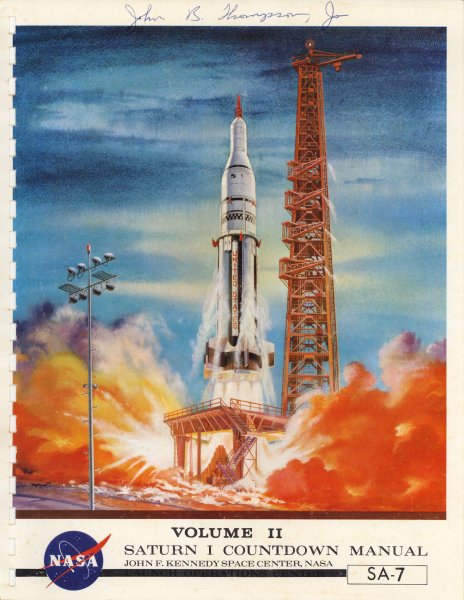The cover of the manual features a detailed hand-drawn illustration of a NASA rocket launching from a large orange scaffolding platform. The white rocket, with “United States” in red text along its side, is depicted with flames and smoke billowing from its base, signifying its imminent takeoff. The background merges shades of blue to resemble the sky, providing a dynamic backdrop to the scene. The rocket's tip is red, with alternating red and black segments along its midsection, complemented by black-and-white checkered triangles.

The border of the manual is a tannish white color, with a white spiral binding evident on the left side. At the top of the border, in blue cursive text, it reads “John F. Kennedy,” followed by a possible cursive signature. The bottom of the border contains black text that reads, “Volume 2, Saturn 1 Countdown Manual, John F. Kennedy Space Center, NASA, SA-7.” On the left side of this text is the NASA logo, a blue circle with white text outlining the agency’s name. The bottom right features “SA-7” in black text within a boxed area, connected by a black line running horizontally beneath the NASA logo. Fire and smoke effects are artistically rendered around the base of the rocket, colored in vibrant hues of yellow, orange, and red, while the smoke appears in shades of gray, white, and black.